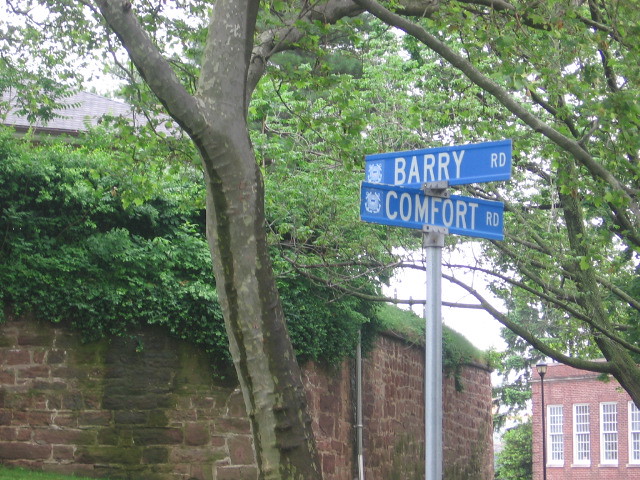In this rectangular, horizontally longer outdoor scene photograph, a stone wall dominates the lower portion, extending from the lower-left to the lower-right, covering approximately three-fourths of the image. Adjacent to this wall on the right side is a building with a deep brick-red hue. This building features four tall, narrow windows with white frames and numerous small panes, situated prominently in its lower right corner. The lush greenery, indicative of a warmer climate, spills over the top of the stone wall in the form of thick brush and shrubs, further complemented by leafy green trees extending from the upper right. A silver street signpost is located at the bottom right of the photo, bearing two blue signs: one displaying "Comfort Road" and, oriented oppositely above it, "Barry Road," both in white text.